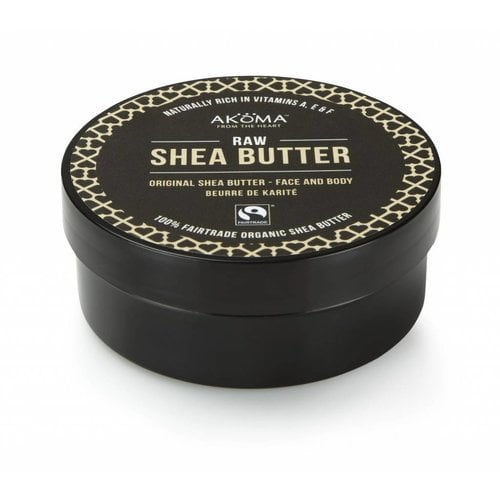The image features a small, circular container of Acoma Raw Shea Butter. The container, which has a twist-open top, is primarily a black or dark brown color and is adorned with a geometric pattern around the perimeter of the lid. The container is described as having a disc shape. The packaging prominently displays multiple inscriptions in white and beige fonts. The top of the container reads "Acoma, from the heart," along with "naturally high in vitamins A, E, and F." Further text includes "original shea butter, face and body," and "Beurre de Karité," emphasizing that it is 100% fair trade organic shea butter. The overall design, which resembles barbed wire or a geometric print, reflects an aesthetically pleasing and thoughtful presentation for the product inside.